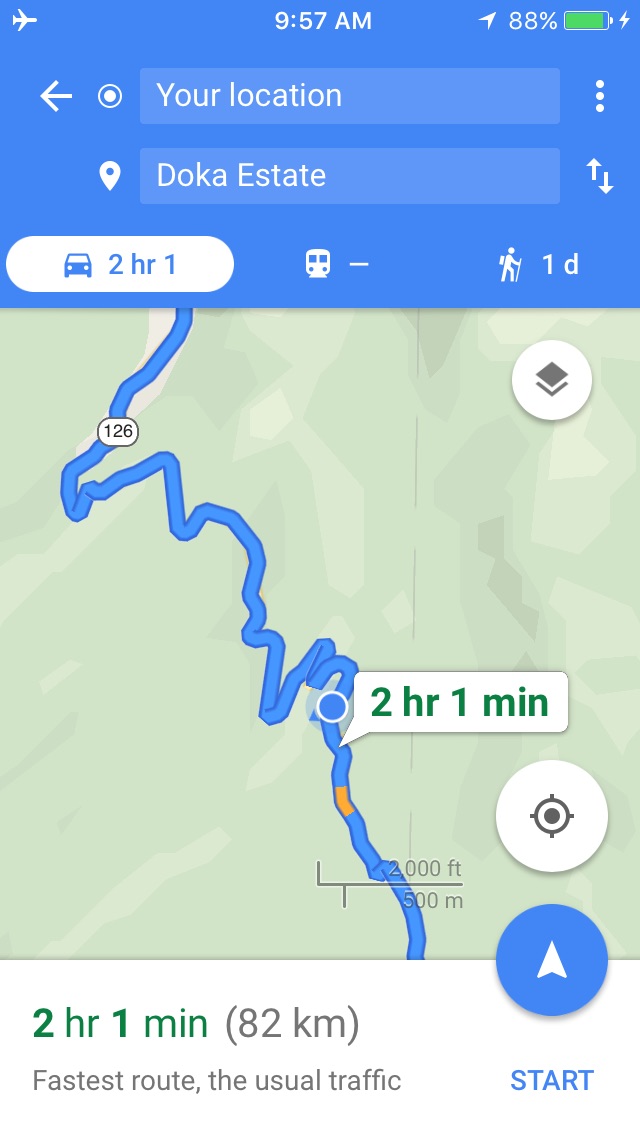The image depicts a cell phone screen displaying a Google Maps navigation interface for a trip to Doka Estate. The detailed map shows an 82-kilometer route primarily via Highway 126, highlighted in blue against a green background. The travel time is estimated at two hours and one minute, deemed the fastest route considering usual traffic conditions. The route includes a segment marked in orange, suggesting a minor delay. The blue line originates from a blue dot indicating the current location. Additional features include buttons to start the navigation and options for different travel modes (including walking and potentially bus routes). At 9:57 a.m., the phone shows 88% battery life and is in airplane mode. The top of the screen displays the travel duration, the intended destination, and battery status.